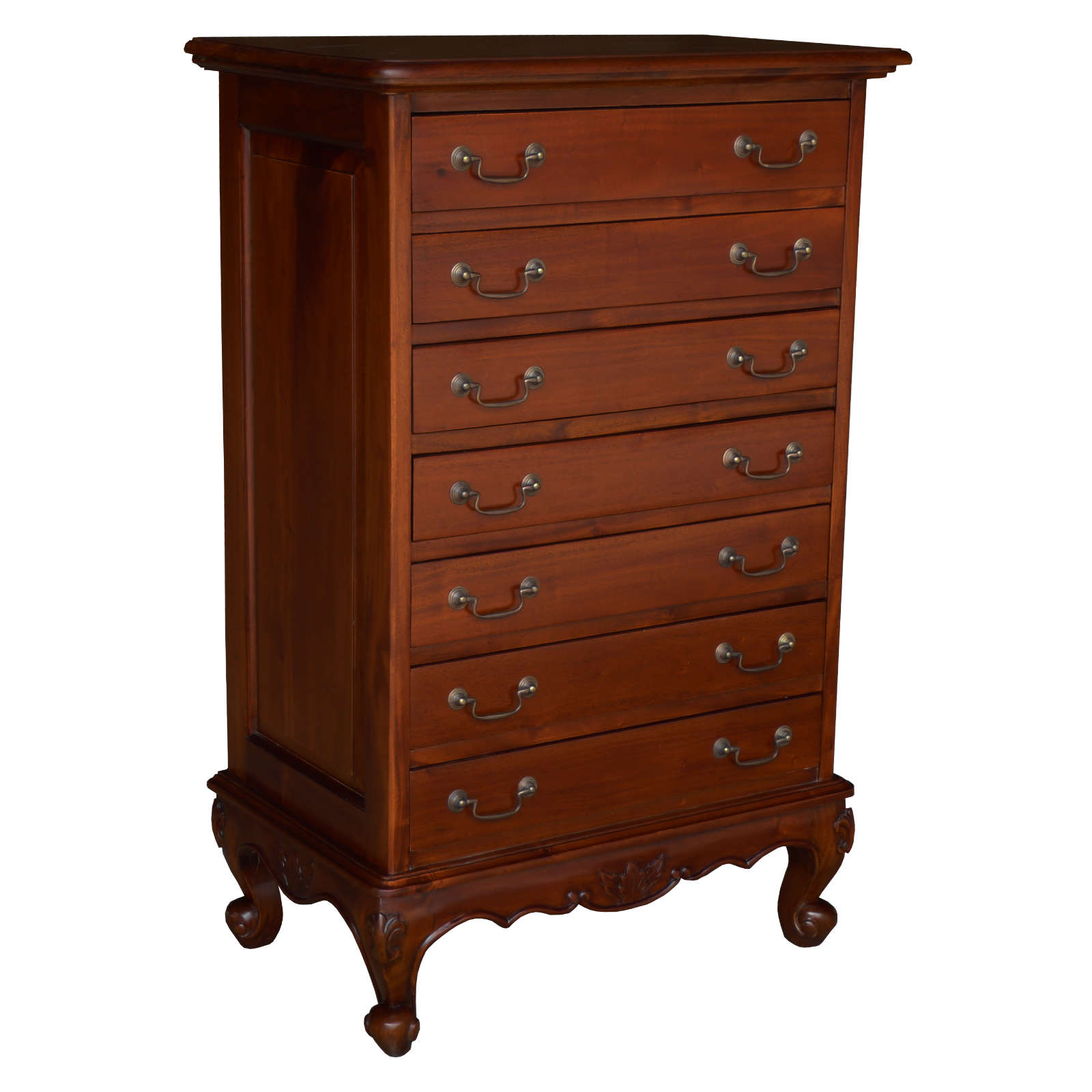The image features an antique wooden dresser, likely from the 1950s or 60s, set against a plain white background with no visible borders. The dresser, constructed from a reddish cherry wood and painted a rich brown color, stands about five inches high and three inches wide, with the front measuring approximately an inch and a half wide and the more visible left side an inch wide. It boasts seven small drawers, each adorned with two silver metal handles on either side. The top surface of the dresser is flat and slightly darker in shade, while the bottom features raised, ornately carved legs, with three visible in the image—two on the left side and one on the front right. Notably, there's a portion in the middle of the bottom that curves outward. Additionally, the left side has a darker, almost black area near the top, adding to its antique charm.